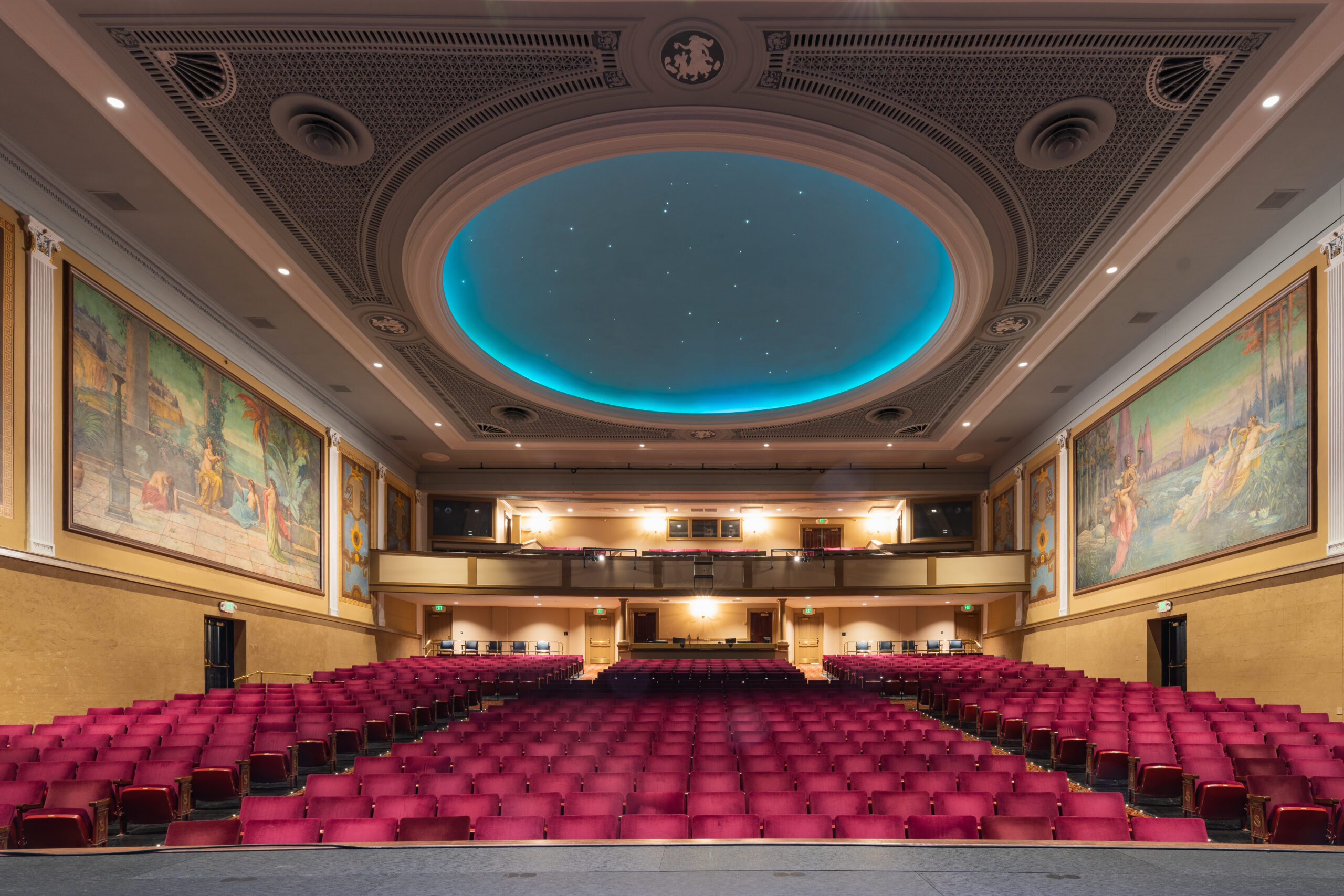This image captures a large, grand theater viewed from the stage, highlighting its opulent and intricate design. The theater boasts an array of purple velvet seats, each row meticulously arranged to accommodate what appears to be an audience capacity of at least 500 to 800 individuals. The seats are plush and stretch across the vast expanse of the auditorium. Flanking the seating area, the walls are adorned with elegant, old-style Renaissance paintings, depicting women in flowing gowns engaging in leisurely activities such as reclining on love seats and being served grapes. These exquisite paintings lend a classic and refined atmosphere to the space.

Nestled toward the rear of the theater is a balcony section, which provides an elevated vantage point for additional seating. Adding to the theater's grandeur are the various lights strategically positioned at the back, illuminating the massive dome-shaped ceiling. This dome features a stunning depiction of a night sky, with specks of white stars twinkling against a dark blue backdrop. The dome itself is accentuated with a baby blue outline, further enhancing its celestial appearance. The walls also feature two emergency exit doors, subtly integrated below the paintings. Amidst the technical setups and seating arrangements, the theater emanates an ambiance of historical elegance and modern functionality.